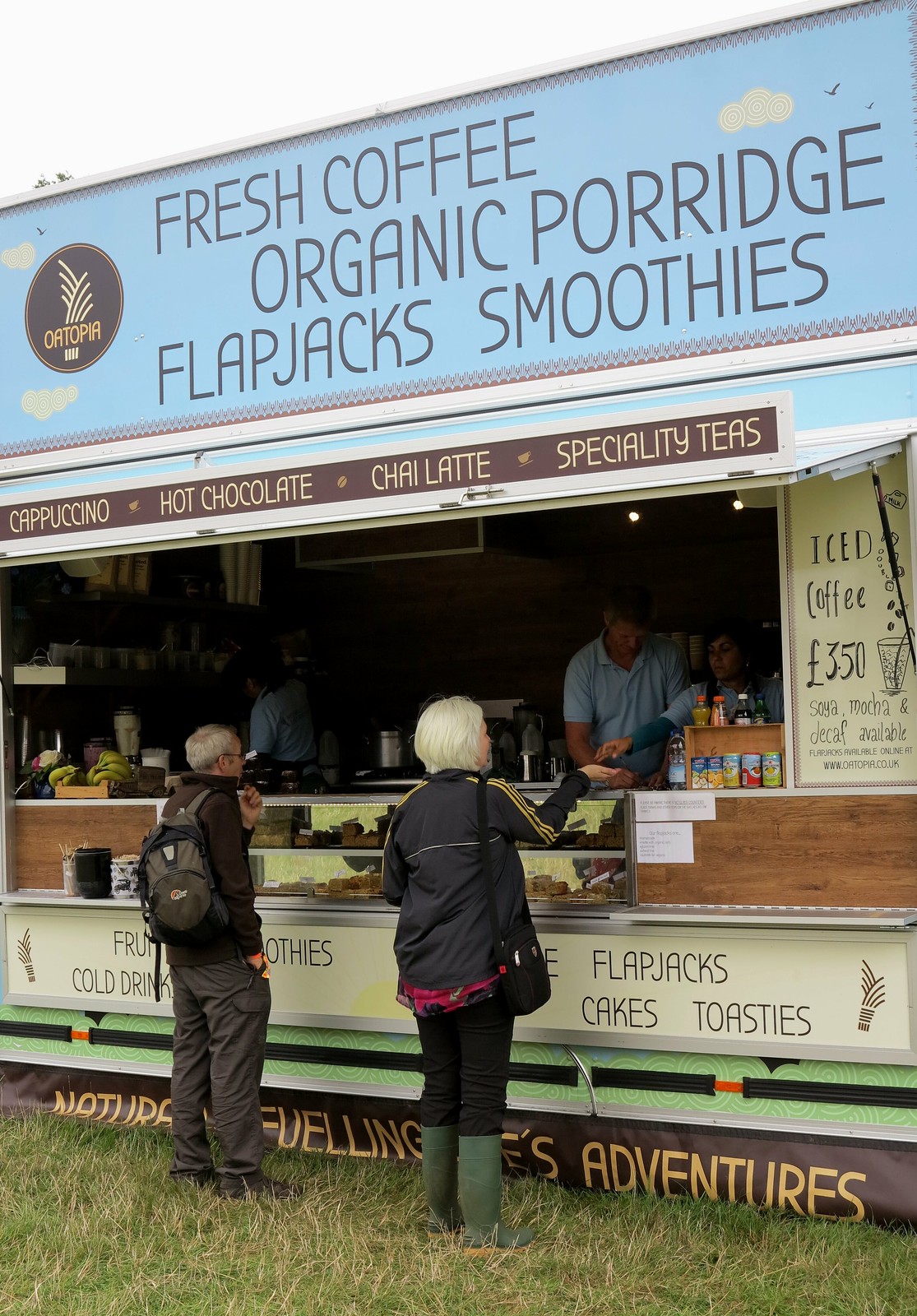In this vibrant outdoor photograph, a bustling mobile coffee stand named "Oatopia" is vividly captured. The stand, which offers an array of items including fresh coffee, organic porridge, flapjacks, smoothies, lattes, hot chocolates, cappuccinos, specialty teas, chai lattes, and iced coffee, is set up on a grassy area, emphasizing its place in a natural setting. The stand features a striking blue sign with brown text and a banner at the bottom reading, "Nature's Fueling Adventures."

Three employees, dressed in blue short-sleeved collared shirts, diligently serve customers. Two of them are engaged in the front, attending to a warmly-dressed older man with a backpack and a woman who appears to be receiving change. The third employee is visible working in the back. A variety of food items are attractively displayed in a front case, drawing the attention of the customers.

The overall scene is a charming blend of warm interaction and tempting offerings, framed within a vertical shot that highlights both the service area and the customers, capturing the essence of a bustling out-of-doors food kiosk dedicated to wholesome and organic products.